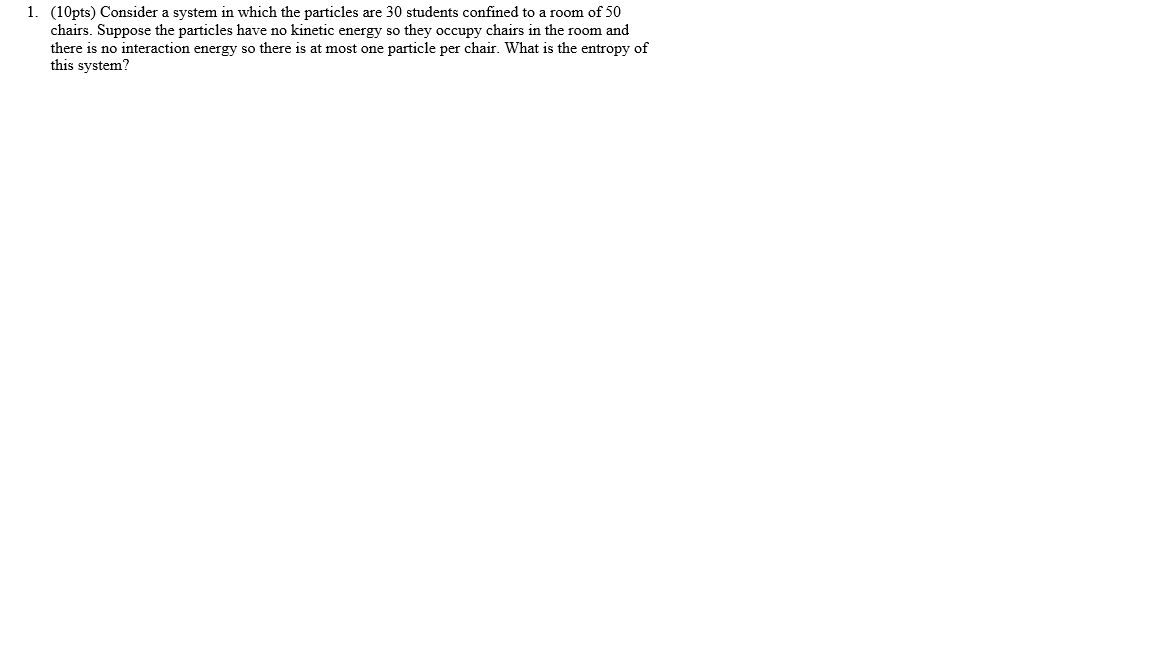A screenshot of an examination page with a completely white background and black text. The text, resembling Times New Roman font in small characters, features a single paragraph positioned at the top of the screen. The paragraph is formatted as follows: "1. (10 pts) Consider a system in which the particles are 30 students confined to a room of 50 chairs. Suppose the particles have no kinetic energy, so they occupy chairs in the room, and there is no interaction energy, so there is at most one particle per chair. What is the entropy of this system?" This appears to be a question extracted from a physics examination. The rest of the screen remains blank.